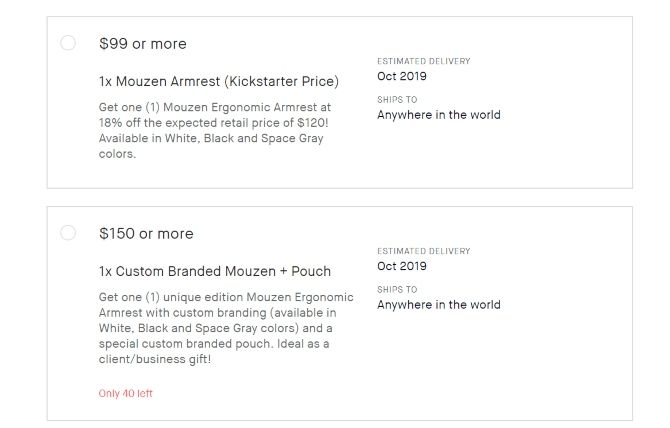The image appears to be a screenshot of a pricing or information page, likely related to a crowdfunding campaign or product listing. The background is predominantly white with text and features two rectangular boxes arranged in a landscape orientation.

**Top Box:**
- **Button:** Located on the left side, appears circular.
- **Price:** Listed as "$99 or more."
- **Description:** "One times museum armrest. Kickstarter price."
- **Estimated Delivery:** "October 2019."
- **Shipping:** "Ships to anywhere in the world."

**Bottom Box:**
- **Button:** Located on the left side, appears circular.
- **Price:** Listed as "$150 or more."
- **Description:** "One times custom branded museum plus pouch."
- **Availability:** "Only 40 left," highlighted in red at the bottom.
- **Estimated Delivery:** "October 2019."
- **Shipping:** "Ships to anywhere in the world."

Both boxes share a similar layout and format, providing concise information about the items, their pricing, and delivery details.